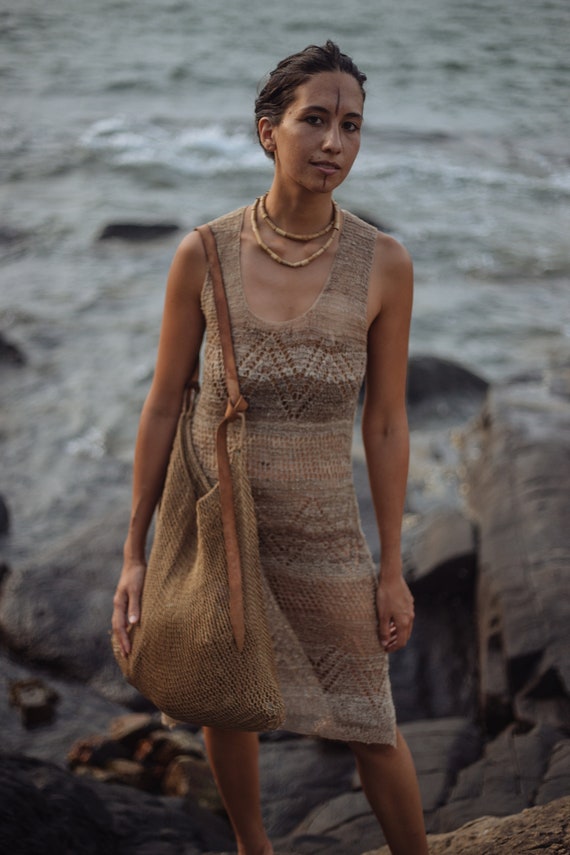The photograph depicts a woman, possibly of Indian or Native American descent, standing in front of what appears to be light gray rock, resembling either a mountainside or a cave, with the hint of a possible carved doorway. She is attired in a woven, tank top dress featuring stripes and zigzag patterns in various shades of brown and gray, embellished with a "W" design made out of brown dots at the chest. The dress has thick straps that go over her shoulders. Her dark brown hair is pulled back into a ponytail, and her makeup includes a distinct vertical black line on her forehead and another running down from below her lips to her chin. She adorns her neck with two necklaces crafted from wooden cylinders; the longer one hangs down into the cut of her dress, while the shorter one sits at the base of her neck. In her right hand, she holds a woven fiber bag with a tan leather strap, slung over her right shoulder and tied in a knot at the front. Her right arm rests on this bag, and her left arm hangs naturally by her side. She gazes directly into the camera, her darker brown skin illuminated gently in the natural light. The background hints at the edge of a body of water, adding a serene, yet rugged, ambiance to the scene.